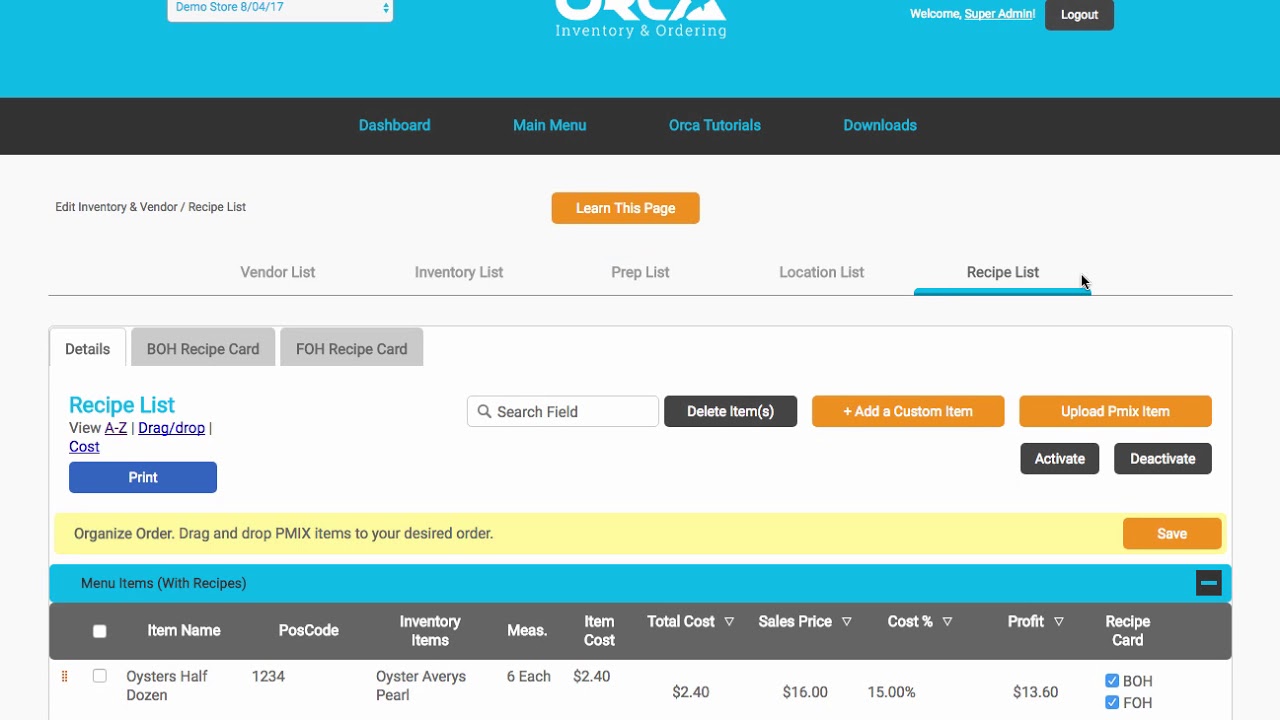The image features a detailed screenshot of a web page dedicated to inventory management and ordering. At the very top of the page, large bold text likely represents the company's name, although it is partially obscured. Directly beneath this, a black rectangular button labeled "Logout" is prominently displayed.

Below the header, the interface is sectioned off, with the main menu options encompassing various functionalities. The first black rectangular button, labeled "Dashboard," is written in blue text. Other menu items, also in blue text, include "Main Menu," "Orca Tutorials," and "Downloads," followed by "Edit Inventory" and "Vendor Receipt List."

Further down, an orange button marked "Learn This Page" in white text stands out. Subsequent lists enumerate different aspects of inventory and management, such as "Vendor List," "Inventory List," "Prep List," "Location List," and "Recipe List."

Underneath these lists, a section titled "Details" highlights "Recipe List." Adjacent to this is an option to "Print." In the same line, additional functions are available including "Delete Items," "Edit Customer Item," and "Upload P-Mix Item" in orange text, except for "Delete Items," which is in black.

On the same line, a black rectangular button with white text provides the options to "Activate" and "Deactivate" items. Finally, at the bottom of the display, a list labeled "Menu Items with Recipes" categorizes various menu-associated recipes.